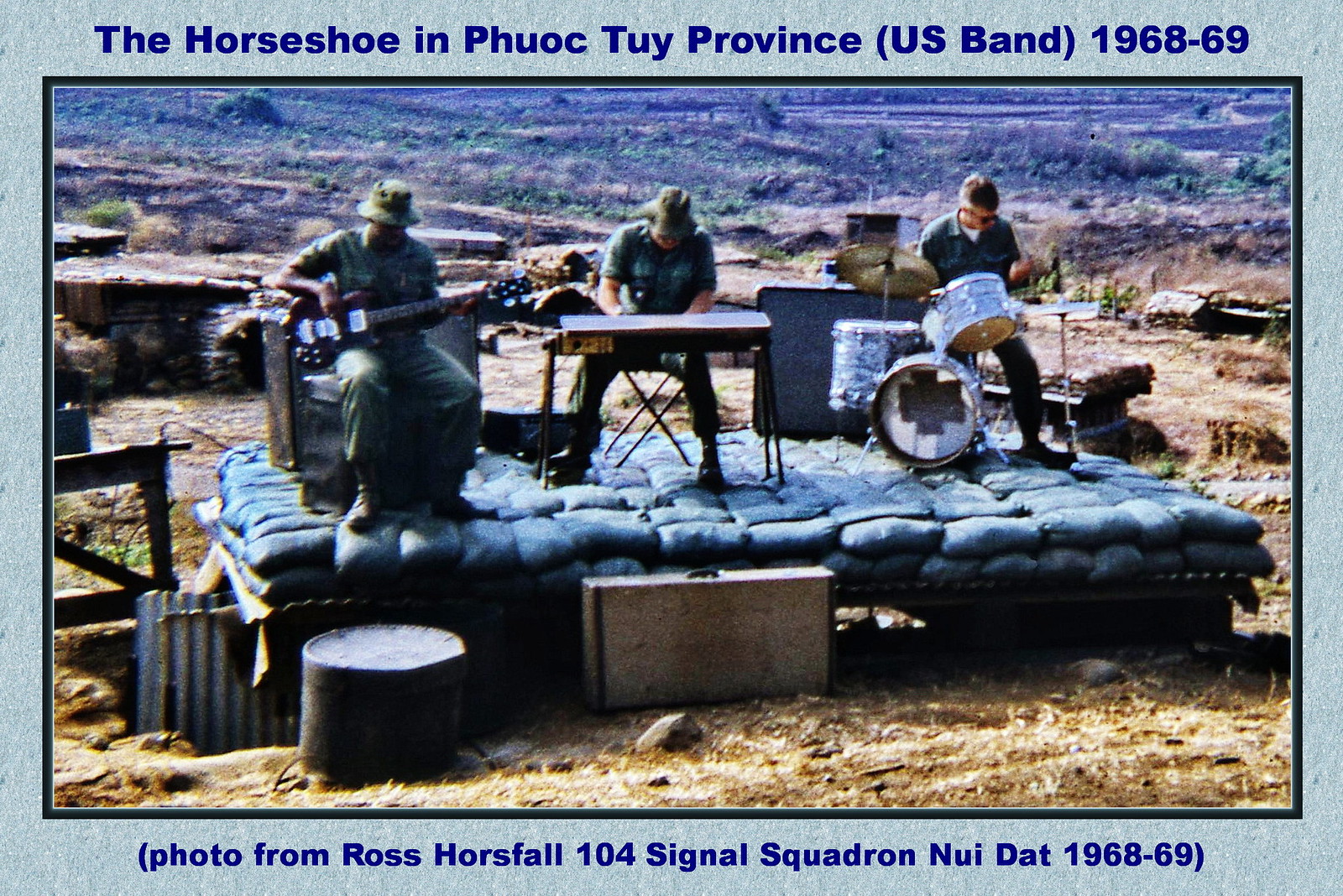This vintage colored photograph captures an outdoor musical performance set against a rugged, uninhabited mountainous landscape. On a raised, cushioned platform, three uniformed performers—donning matching green outfits and hats—are poised in the midst of their concert. The leftmost musician, seated on what appears to be a sofa, strums a guitar. At the center, another performer is engrossed in playing a keyboard, while the rightmost individual skillfully handles the drums. Behind them, a black screen provides a stark backdrop.

On the left edge of the image, remnants of broken huts can be observed, along with some cylindrical drums and a centrally positioned trunk-like box. The picture is framed with a black border and set against a light blue background. At the top, the caption reads: "The Horseshoe in Puyolk, Tu Province, (U.S. Band, 1968-69)." A footnote at the bottom credits the photo to Ross Horsfall from the "104 Signal Squadron, New Datt, 1968-69."